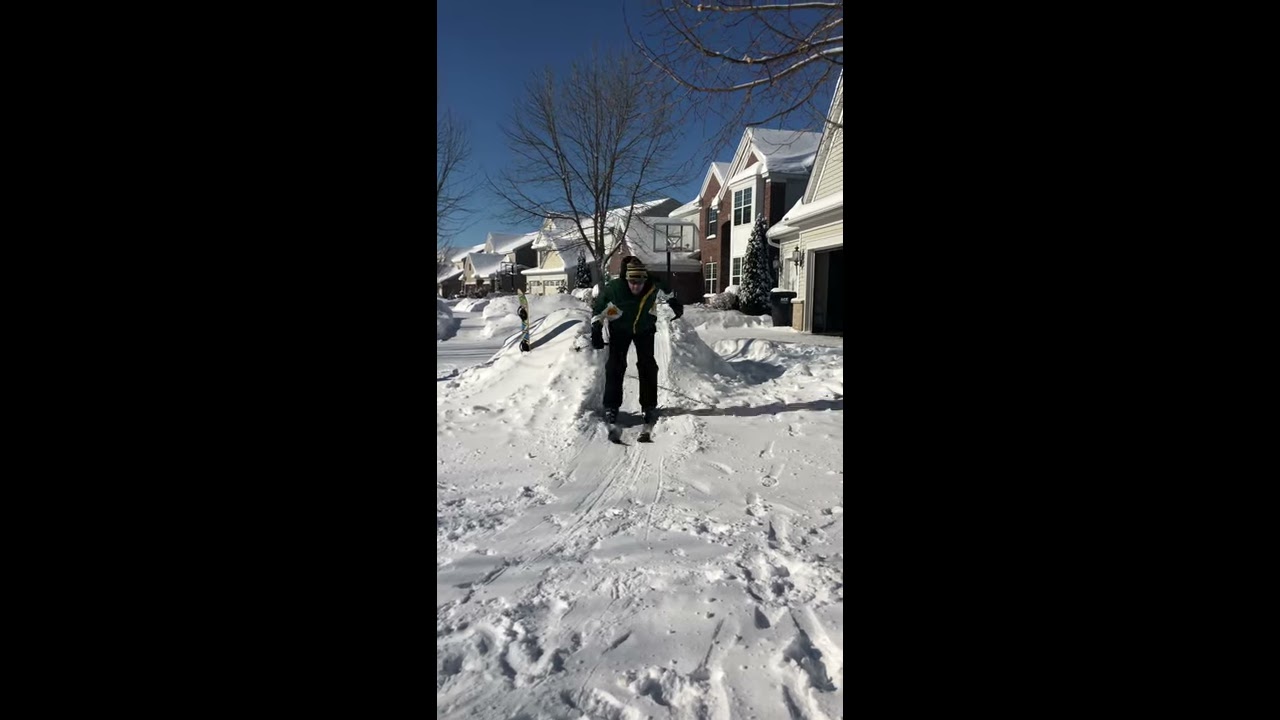A person wearing a black winter snowsuit and a beanie is skiing down a small snow mound in the front yard of a residential area. The skier stands out prominently against the pristine, white snow, which is dotted with tracks and footprints. In the background, there is a row of two-story houses. One house has a basketball net visible, and the roofs are covered in snow. The houses are a mix of white, brown, and dark gray. The blue sky above is partly obscured by the bare branches of deciduous trees, allowing the clear sky to peek through. The image has a wide black border on both sides, giving it a vertical, cell phone-style appearance.